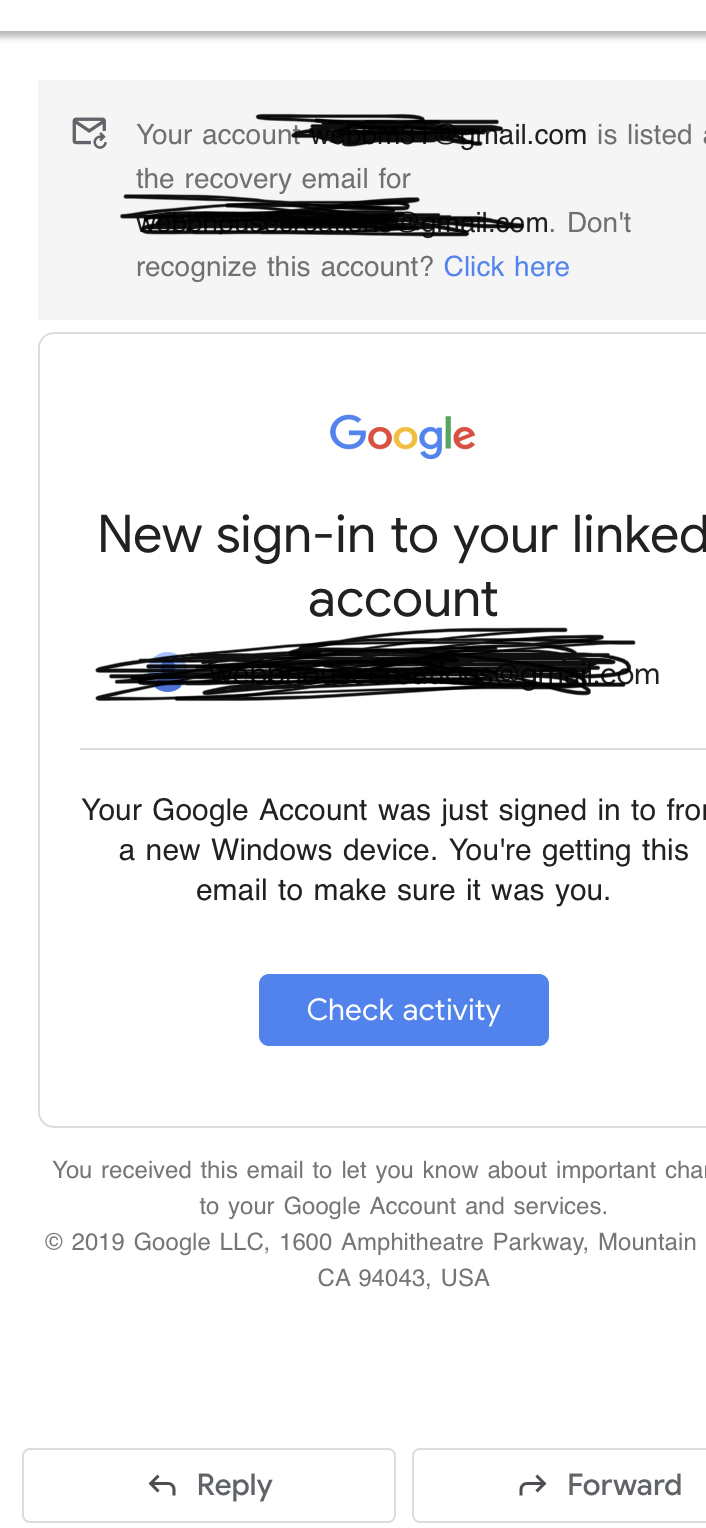This image appears to be a screenshot of an email viewed on a mobile device. The email has three distinct areas obscured with black scribbles to obscure sensitive information. At the top is a gray rectangle, containing an envelope icon and the partially hidden text "Your account," followed by a Gmail address that has been largely blacked out, showing only "mail.com." Below, text indicates "The recovery email for" another similarly scribbled-out email address, ending in "gmail.com." There’s a line saying "Don't recognize this account?" followed by an actionable phrase in blue text, "Click here."

Beneath the gray section, the background turns white. The header features the Google logo in its signature multicolored style. Further down, it informs the recipient of a "New sign in to your linked account," which has also been scribbled out but is indicated to be a Gmail account. The email alerts the recipient that their Google account was accessed from a new Windows device, aiming to ensure that this activity was authorized. The email includes a blue button labeled "Check activity" for the recipient to verify the sign-in details. Lastly, the bottom of the email has standard options to "Reply" on the left and "Forward" on the right.